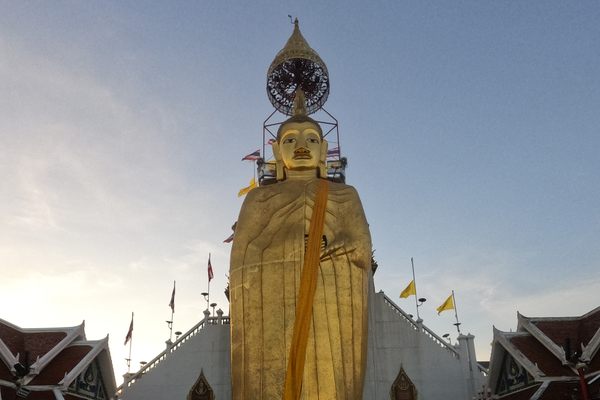This photograph captures an extremely tall and majestic gold statue of a man, featuring elements suggestive of Buddha or a significant Asian figure, possibly Confucius. The statue, adorned with earrings and a detailed headdress or apparatus, towers several stories high, its grandeur emphasized by the clear blue sky and scattered clouds in the background. Above its head, an intriguing, almost moon or teardrop-shaped structure is suspended, connected to the statue by several poles from the back. The statue stands in front of a double-set staircase—with steps on both the left and right—leading to its base. Surrounding the statue are various buildings, possibly houses, partially obscured. Flags, including noticeable yellow ones and possibly reddish ones, are scattered along the stairways, swaying gently in the outdoor setting, which appears to be set in daylight. The entire scene presents a mix of natural and surreal elements, amplifying the statue's imposing presence.